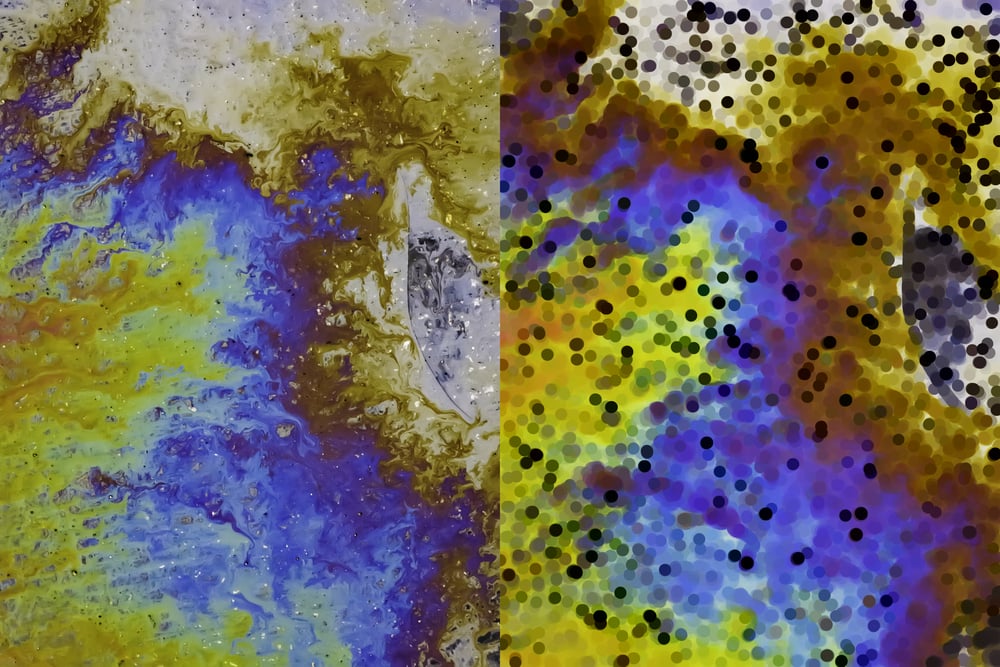This image features a side-by-side comparison of two art pieces. On the left, the painting is fully revealed, showcasing a dynamic landscape. A blue waterway runs through the middle, surrounded by yellow flame-like patterns to the left and right, creating a striking contrast. The background has a cracker-like texture interspersed with white, brown, and ivory hues, contributing to a rich, tactile quality. 

On the right side, the same painting is pixelated and blurred, transforming into an abstract mosaic of colors. Brown, tan, green, blue, ivory, and black pin-dot patterns cover the entire image, resembling tiny beads dispersed throughout the art. The transition from the clear, defined artwork on the left to the dotted, pixelated version on the right highlights the intricate details that compose the overall texture and tonality of the painting.